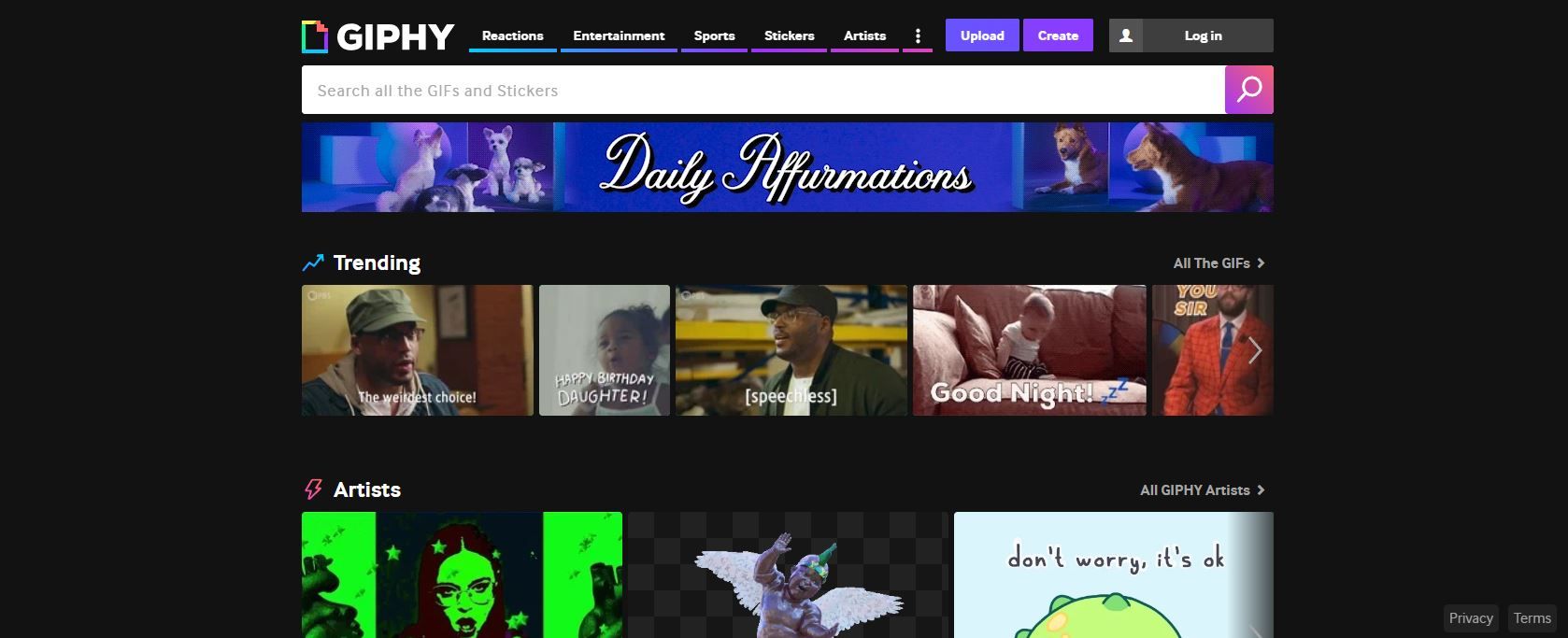The image captures a screenshot of the Giphy homepage, with a predominantly black background. At the top of the screen, the Giphy logo, spelled "G-I-P-H-Y," is prominently displayed. The header includes several navigation options: "Reactions," "Entertainment," "Sports," "Stickers," "Artists," an "Upload" button, and a "Create" button. Additionally, there is an icon resembling a silhouette of a person, implying a profile or account access point, and a "Log In" section.

Below the header, a large, white search bar spans nearly the entire width of the screen, prompting users to "Search all the GIFs and stickers." 

Underneath the search bar, various rows of GIFs are displayed. The top row showcases different animals, while the row below features diverse people and is labeled "Trending." 

In the center of the screen, a section titled "Daily Affirmations" is highlighted, with text in cursive white font set against a royal blue background.

The bottom part of the screen includes a section labeled "Artist," which appears to spotlight various Giphy artists. To the right, there is another section titled "All GFs," showcasing a broader range of GIF content.